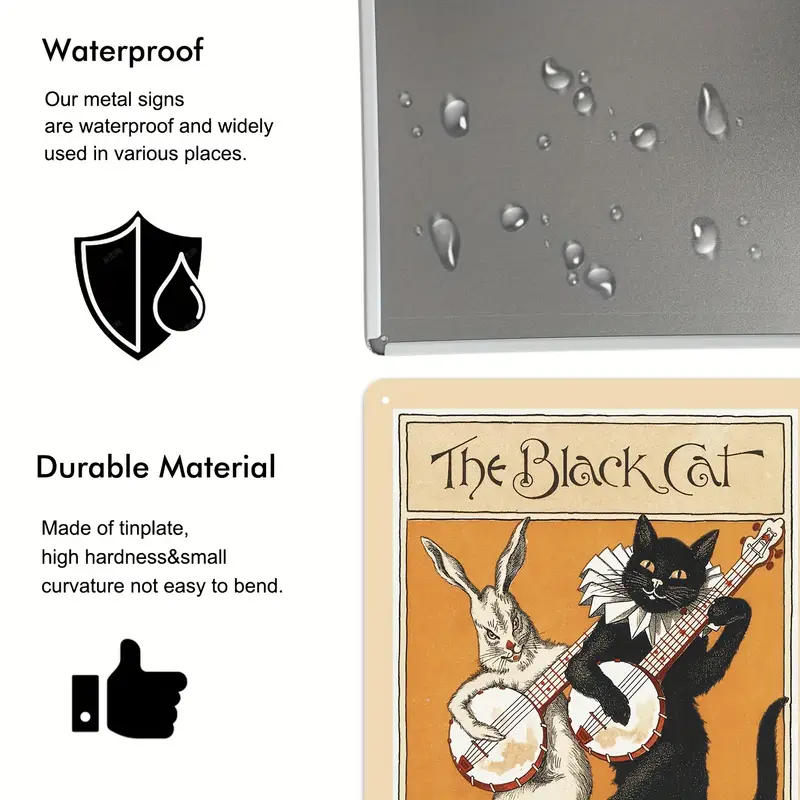The image consists of two sections with symbols, icons, and text. On the left side, starting from the upper left corner, bold black text states "Waterproof." Below this, left-aligned text explains, "Our metal signs are waterproof and widely used in various places." Adjacent to the text is a black shield outlined in white, featuring a similar-styled water droplet on the right side. In the lower left corner, bold text announces "Durable Material." The subsequent left-aligned text reads, "Made of tin plate, high hardness, and small curvature, not easy to bend," beside a black outlined thumbs-up icon.

On the upper right side, an image depicts a square, dark gray or silvery surface adorned with multiple water droplets, demonstrating its waterproof quality. In the lower right corner, there’s a sign titled "The Black Cat," featuring a whimsical illustration of a cat and a bunny playing banjos, complete with a hole in the upper left corner for hanging.